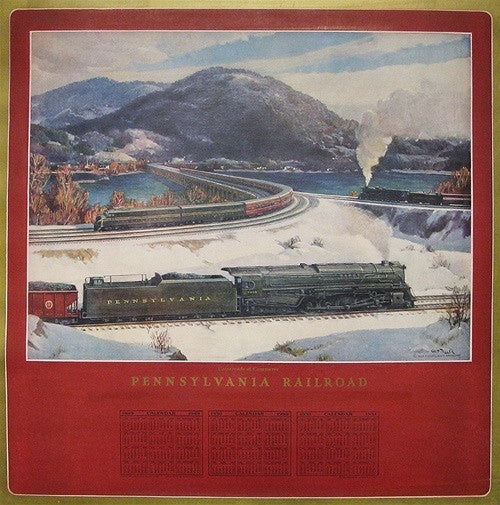This is a detailed depiction of a vintage-style calendar poster featuring a scenic railway illustration. Framed with a brownish-green border and set against a red background, the top of the poster showcases a painting of three black steam engine trains running on three separate tracks through a picturesque snow-covered landscape. The central train emits a significant amount of smoke. Surrounding the tracks, there are serene snow-covered hills, a water body, rugged gray mountains, and a blue sky adorned with white clouds. Below this vivid winter scene, the text "Pennsylvania Railroad" is prominently displayed in golden capital letters. Beneath this heading, a practical timetable chart is presented, likely indicating the calendar months and days in black and gold text. The overall composition vividly encapsulates a railway scene in a snowy, mountainous environment, blending functionality with artistic charm.